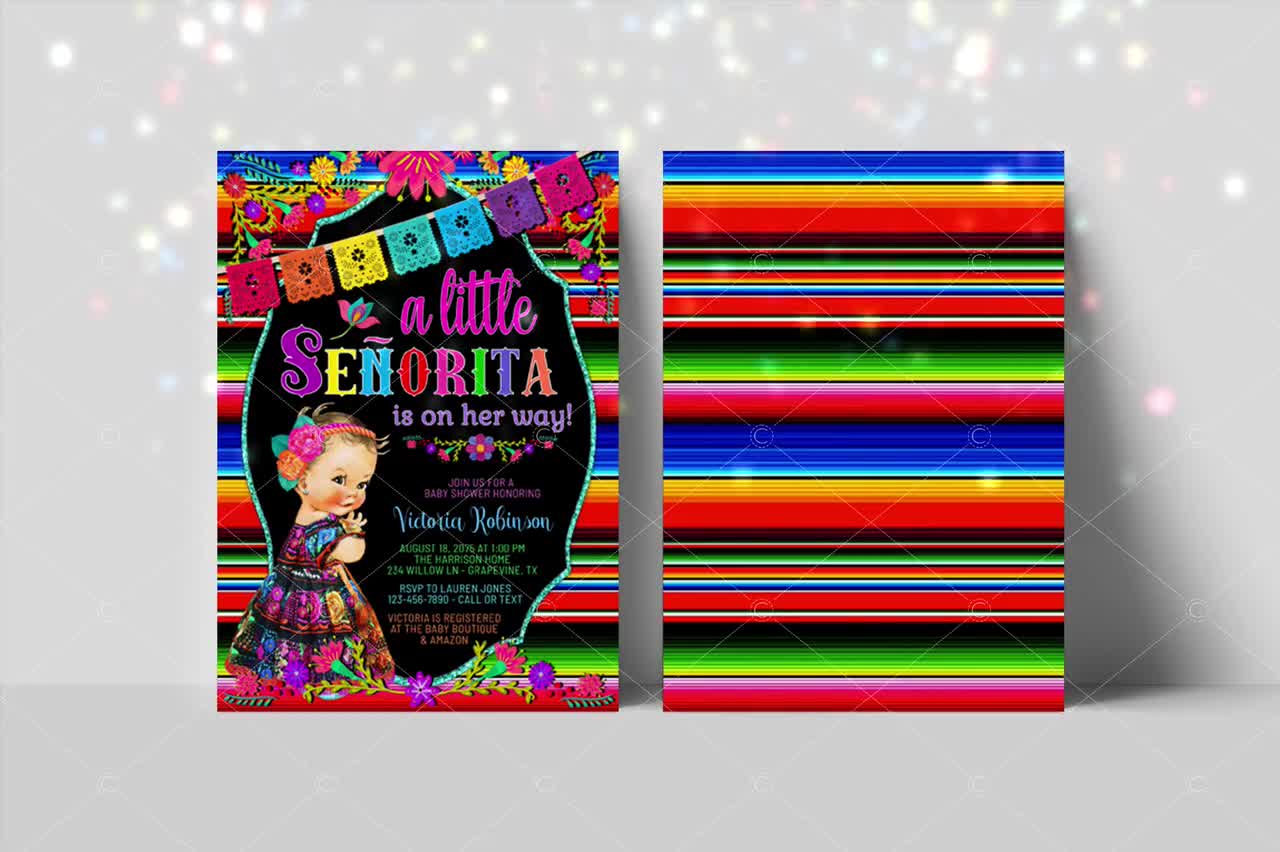This is a detailed image of a baby shower invitation. The vibrant background features horizontal stripes in shades of red, green, fluorescent green, blue, and more, separated by small black lines. A string adorned with colorful paper flags in hues of red, orange, yellow, teal, blue, purple, and pink extends across the top. Both the header and footer of the invitation are elaborately decorated with bright flowers, incorporating colors like purple, pink, and orange. 

The focal point of the invitation is a black shield-shaped section framed by a green border, which houses the main text. In colorful fonts, it announces, "A little señorita is on her way." Adjacent to this, there is an illustration of a little girl. Below, it reads, "Join us for a baby shower honoring Victoria Robinson. August 18, 2023 at 1 p.m. The Harrison Home, 234 Willow Lane, Grapevine, Texas. RSVP to Lauren Jones, 123-456-7890-call or text. Victoria is registered at the Baby Boutique and Amazon." Each segment of text is printed in a different vibrant color, contributing to the festive and joyous atmosphere of the invitation.